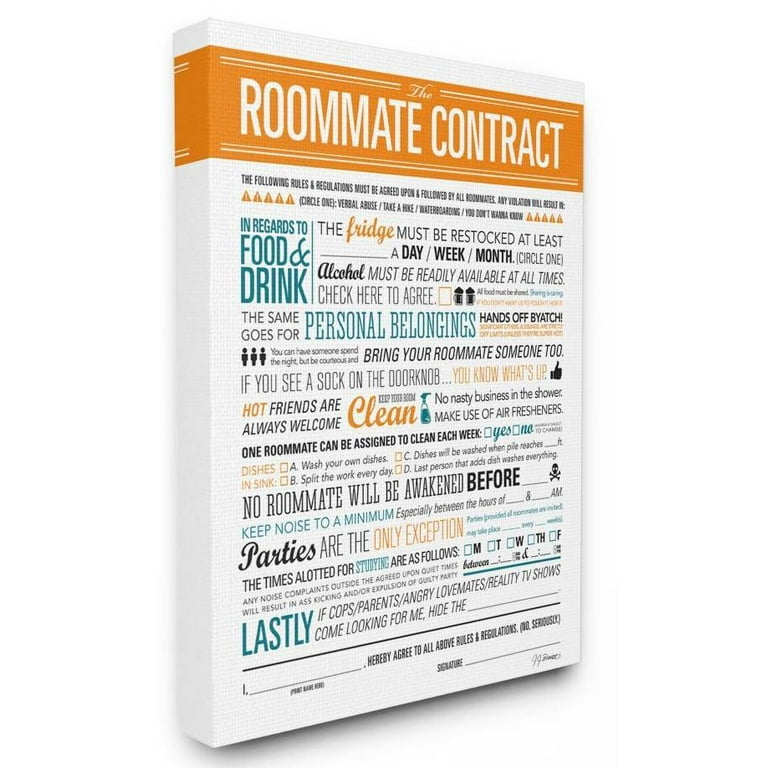The image features a whimsical and humorous "Roommate Contract" displayed on a canvas with white text framed by an orange border, set against a yellow background. At the top, in bold white letters, it reads: "The Roommate Contract." Directly below, the contract stipulates in varied colorful fonts: "The following rules and regulations must be agreed upon and followed by all roommates. Violations result in verbal abuse." This playful document includes several comedic rules, such as provisions for restocking the fridge with the frequency (day, week, or month) to be checked, and an insistence that "Alcohol must be readily available at all times" with a checkbox for agreement.

The left side of the contract humorously addresses personal boundaries with statements like “In regards to food and drink, the same goes for personal belongings: Hands off!” It features a silhouetted trio of figures and adds, “Bring your roommate someone too,” along with the cheeky note in red, “If you see a sock on the doorknob, you know what’s up.” The contract further mandates cleanliness with rules about avoiding “nasty business in the shower” and regular use of air fresheners, suggesting that cleaning duties can be assigned weekly with a “Yes / No” option.

Additional rules specify that no roommate should be awakened before a set time, except for parties, and that “The time allotted for studies” should be indicated for different days of the week. The final rule is a pledge to hide a roommate upon inquiry by “cops, parents, angry love mates, reality TV shows.”

At the bottom, the contract concludes with a declaration: "I, [space for name], hereby agree to all the above rules and regulations. No, seriously." Below this, there is a space for a signature, tying together the playful and satirical nature of the "Roommate Contract." The diagonally viewed canvas casts a shadow to the right and bottom, adding a touch of depth to the image.